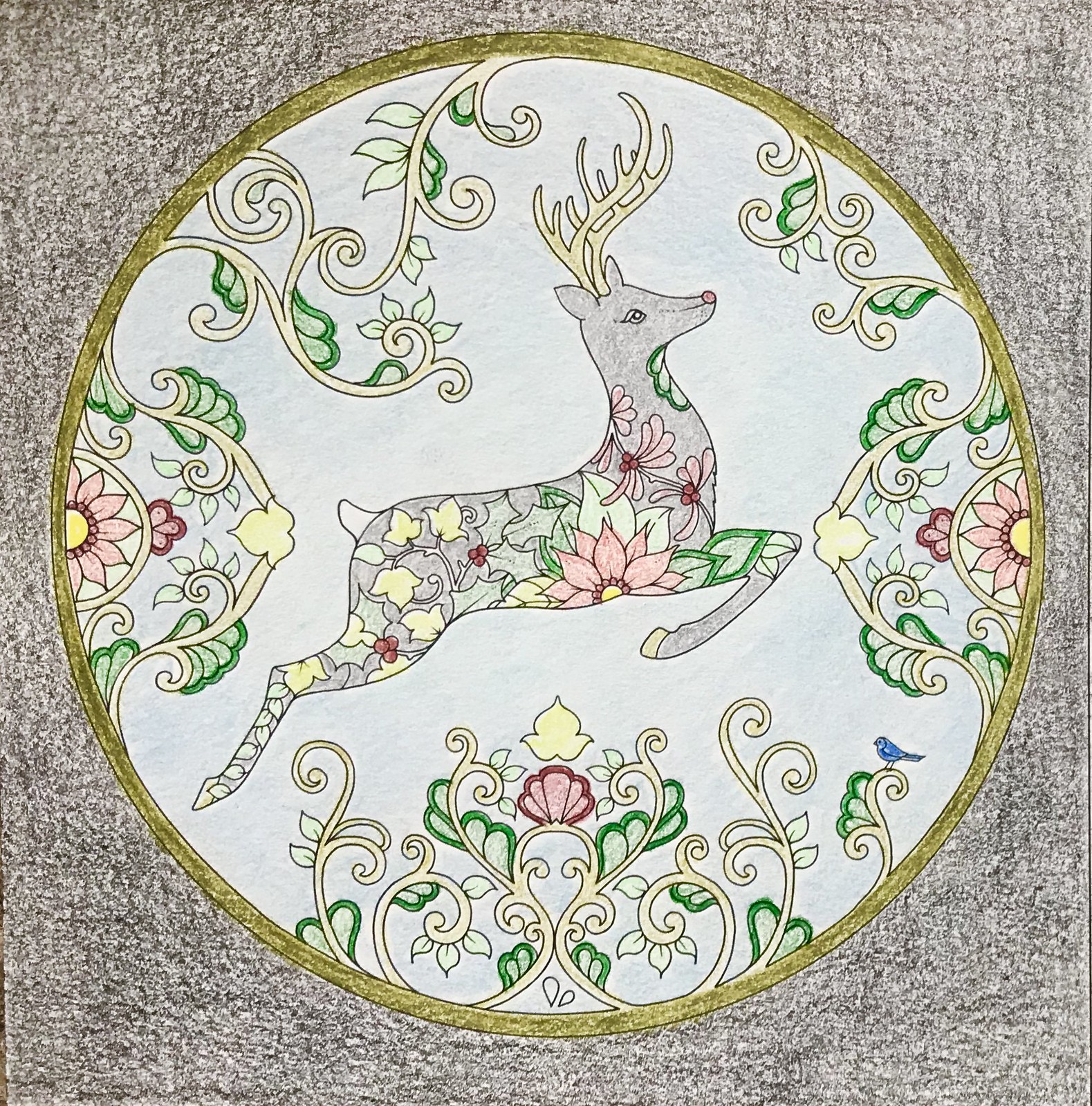The image is a digitally scanned, hand-drawn and colored illustration, housed within a perfectly square frame. The background texture suggests it was originally created on paper. Dominating the composition is a prominent circle, outlined by a golden circumference border. Inside this circle, the main subject is a leaping reindeer, angled slightly with its head tipping upward towards the two o'clock position. The reindeer's body is predominantly grey, decorated with a profusion of colorful flowers and leaves that seamlessly blend into its form. It has white antlers adorned with additional flowers and vines, and its hooves exhibit yellow hues. A small blue bird is perched near the deer. 

The interior of the circle features a light blue background, while the outer circle is encircled by vines, leaves, and swirling patterns that extend from just inside the golden border. The entire image carries a festive, Christmas-like atmosphere, with red flowers, holly, and decorative swirls enhancing the overall design.